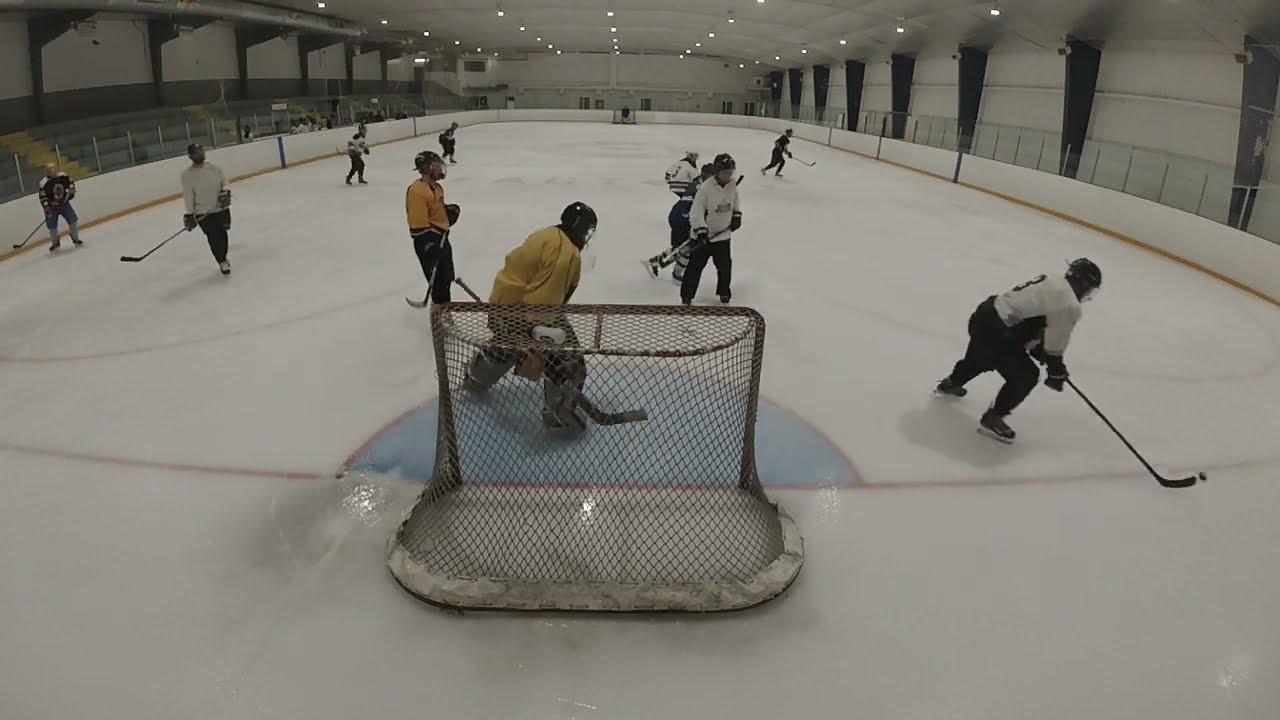This indoor photograph captures a hockey practice session at a small ice rink with a very low roof line. The perspective is from behind a white goal net, looking down the rink towards the other end where two teams are engaged in practice. The rink itself is pristine white with red lines and a distinct blue semicircle around the goalie crease. Surrounding the rink, there are white barriers featuring a yellow stripe along the base, topped with what looks like glass or plexiglass boards.

On the ice, the majority of players wear white jerseys, with a few in yellow and one in black. The goalie at the far end is distinguishable in a yellow outfit with black pants. A white jersey-clad player at the lower right of the image is in control of the puck, planning his next move while the goalie and other players focus on him.

Bleachers, five or six rows high, are located only on the left side of the rink, and they are empty. No bleachers are visible on the other three sides. Blue banners or rafters are positioned intermittently above the rink. Additional players can be seen in the distance in the players' box, potentially including a coach on the sidelines.